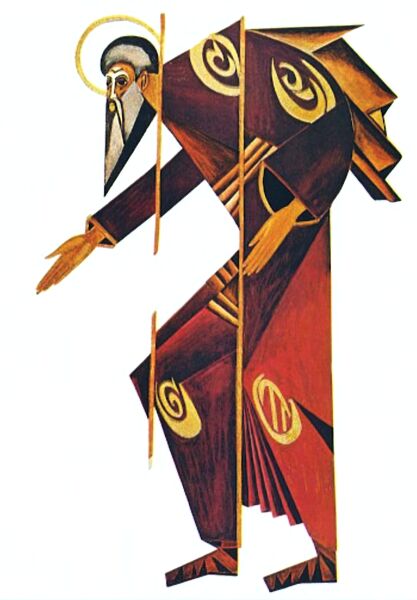This is an angular, two-dimensional marker illustration depicting a religious-looking figure, likely a saint, characterized by sharp, geometric shapes. The man's head features a black outline with gray hair and a long, triangle-pointed beard, framed by a gold halo. His body is segmented horizontally, resulting in a slightly off-centered appearance, with portions of his form misaligned. Dressed in a red and burgundy robe with a gold belt, his attire includes a prominent shoulder designed as a sideways triangle adorned with a yellow circle. His hands and fingers extend forward, elongated and pointed, continuing the angular theme. His knee is notably pointy, and he wears shoes that seem to be bound, also depicted in sharp, triangular forms. The figure's sharp shape and elaborate use of triangles create a striking cubist effect, emphasizing the religious and saintly representation.